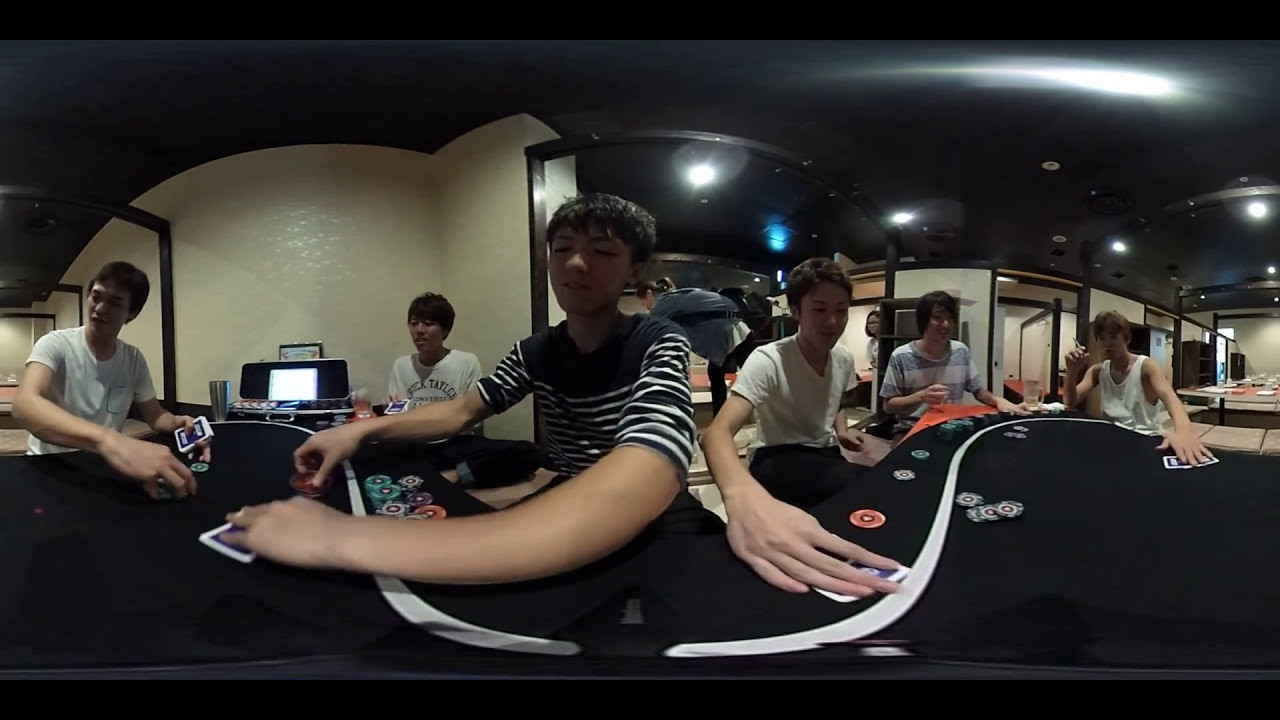In this distorted panoramic image, six Asian teenagers are gathered around a black-and-white poker table, immersed in a game of poker. The table is scattered with colorful poker chips in shades of gray, green, purple, and red, along with several playing cards. Dominating the foreground, the table is central to the composition, with the teenagers seated around it, their hands placed over their dealt cards. Most of them are wearing white shirts, while two boys stand out in striped shirts—one with gray and white horizontal stripes, and another in navy blue with white stripes.

The background features a tan-colored wall, its lines curving bizarrely due to the panorama's distortion. Two additional people can be seen in the blurred background: a woman observing the game from afar and another person with a backpack, stooped over. Some of the teenagers are smiling, while others are deeply engrossed in their cards, creating a lively yet focused atmosphere. Despite the setting suggesting a casino environment, the casual attire and playful engagement of the teenagers imply a friendly, informal game rather than a high-stakes gambling scenario.